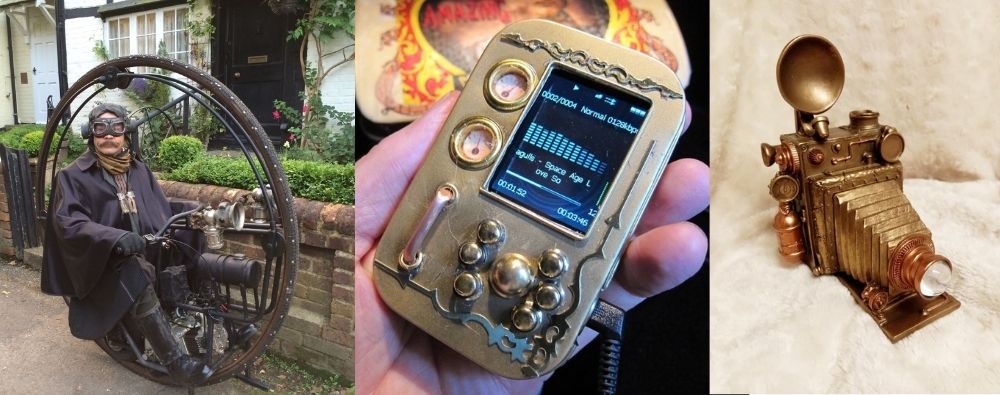A captivating series of three steampunk-themed images is presented in a single detailed scene. On the left, a man is seated in a unique, handcrafted vehicle that appears to be a one-person, large-wheeled motorcycle with a singular circular frame enveloping him. He sports a steampunk ensemble, complete with a black trench coat, knee-high black leather boots, aviator goggles, and a beige bandana, situated in a daytime urban setting adorned with a lined brick wall, green shrubbery, and a white house. The vehicle features a headlight, a small motor near his legs, handlebars, and a prominent horn at the front, suggesting a fantastical fusion of retro-futuristic design and functionality. 

The central image showcases a steampunk-style electronic device resembling an mp3 player. It is silver with a central screen display surrounded by a mixture of round and rectangular dials and gauges, intricate detailing in the form of two round dials, and LED readouts indicating various operational statistics such as internet speed and packet loss, all executed in steampunk aesthetics.

On the right, there is an ornate, brass camera with a large, globular lens positioned on a multi-tiered platform. It features an oversized flash, adding to its grand and elaborate appearance. The camera, reminiscent of antique designs from the 1800s, has been artistically enhanced with gold foil and bronze paint, giving it a distinguished, steampunk-inspired look. Each piece in the series blends functionality with art, creating a vivid representation of steampunk culture.